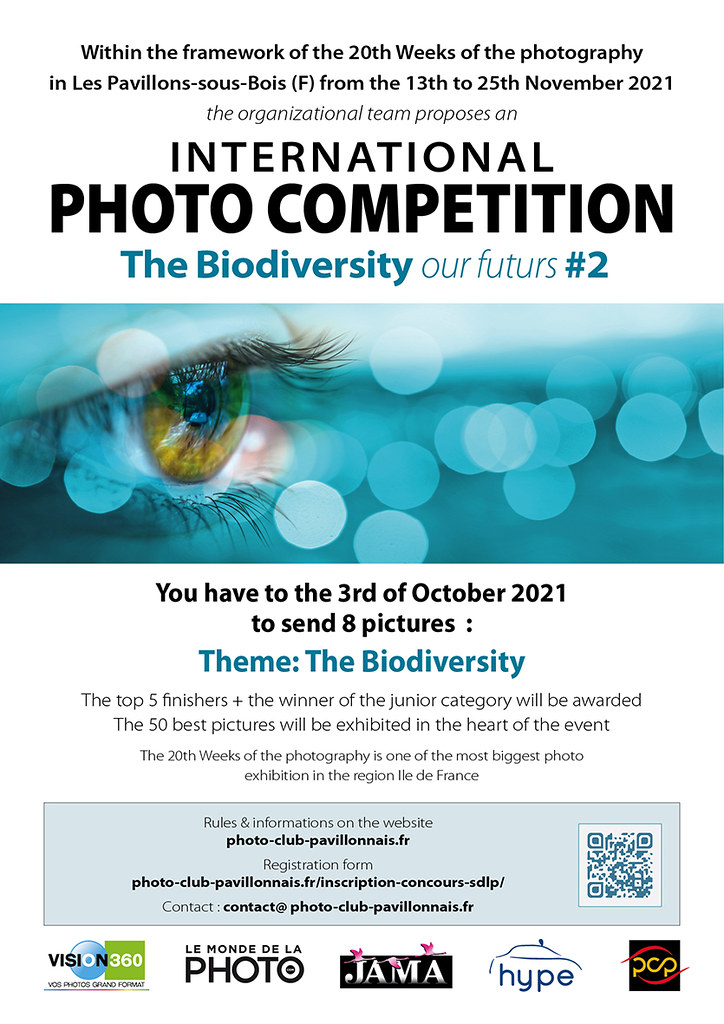The image is an advertisement pamphlet for an international photo competition titled "The Biodiversity: Our Futures" (Number 2). In black text, it provides key information and instructions. The cover prominently features a detailed close-up image of a blue-tinted eye with small blue bubbles in the background. Below the image, it states that participants have until the 3rd of October 2021 to submit a set of eight pictures on the theme of biodiversity. It emphasizes that the top five finishers and the winner of the junior category will be awarded. Additionally, the 50 best pictures will be exhibited as a central feature of the event, which takes place within the framework of the "20th Weeks of Photography" at Les Pavilions, scheduled from the 13th to 25th November 2021. The bottom section of the pamphlet includes advertisements from sponsors and a barcode that can be scanned for more information about the event.